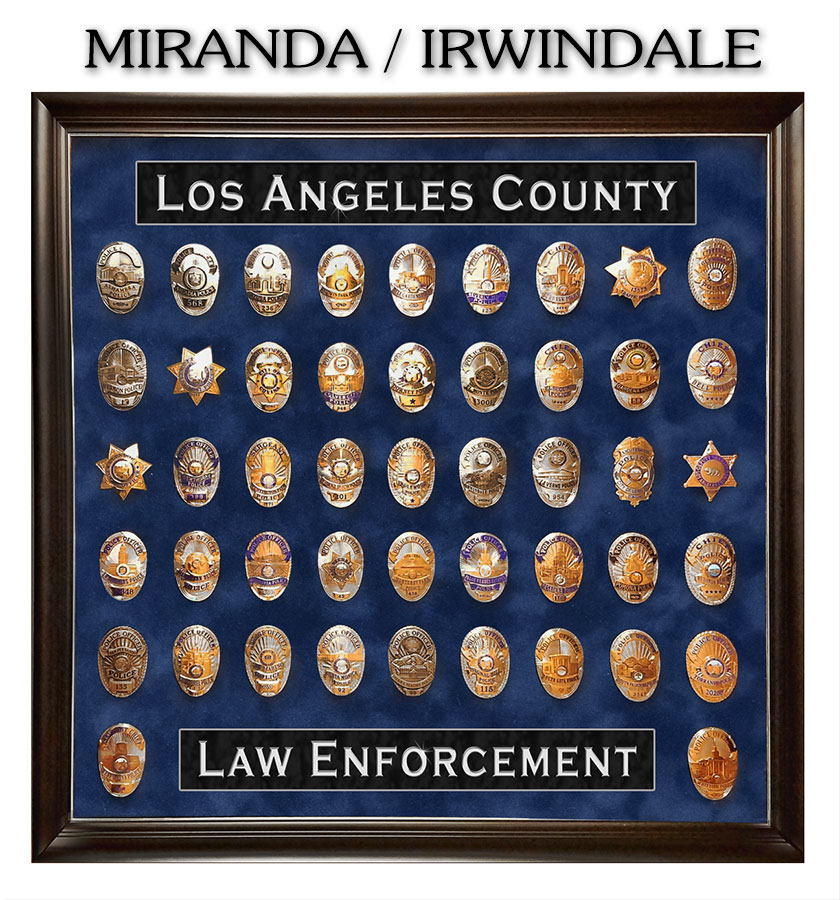This detailed image depicts a meticulously arranged display of approximately 50 law enforcement badges, all framed within a dark brown wooden frame that boasts a blue marbled velvet background. The badges, which vary in shape and color—some oval, some star-shaped, with most adorned in gold and brown hues, and a few featuring blue accents—are neatly organized in five uniform rows of nine badges each. The frame is crowned with a black banner featuring bold white text that reads "Los Angeles County," while a similar banner at the bottom states "Law Enforcement" in all-caps. Just above the main frame, on the white background, the words "Miranda / Irwindale" are inscribed in black font. Additionally, two badges are positioned on either side of the "Law Enforcement" text at the bottom, adding symmetry to the detailed and orderly display.